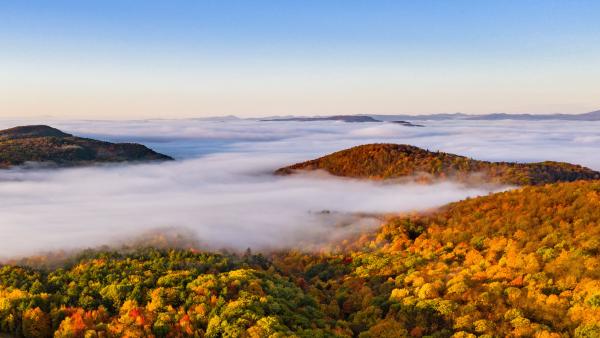A breathtaking landscape image taken from the peak of a mountain captures a vast, awe-inspiring view of rolling hills and distant mountain ranges. The scene is enveloped in a serene mixture of colors, with the sun either rising or setting, casting a warm orange-green hue over the lush, forested terrain. The vibrant foliage showcases an autumnal palette, with leaves in shades of green, yellow, orange, red, and brown. Below the vantage point, a blanket of mist or clouds nestles in the valleys, creating an ethereal layer that contrasts beautifully with the clear, blue sky above. The image presents a layered composition where the tops of several hills and mountains pierce through the mist, accentuating the depth of the landscape. The horizon reveals more mountain peaks, further emphasizing the untouched beauty of this mountainous vista.